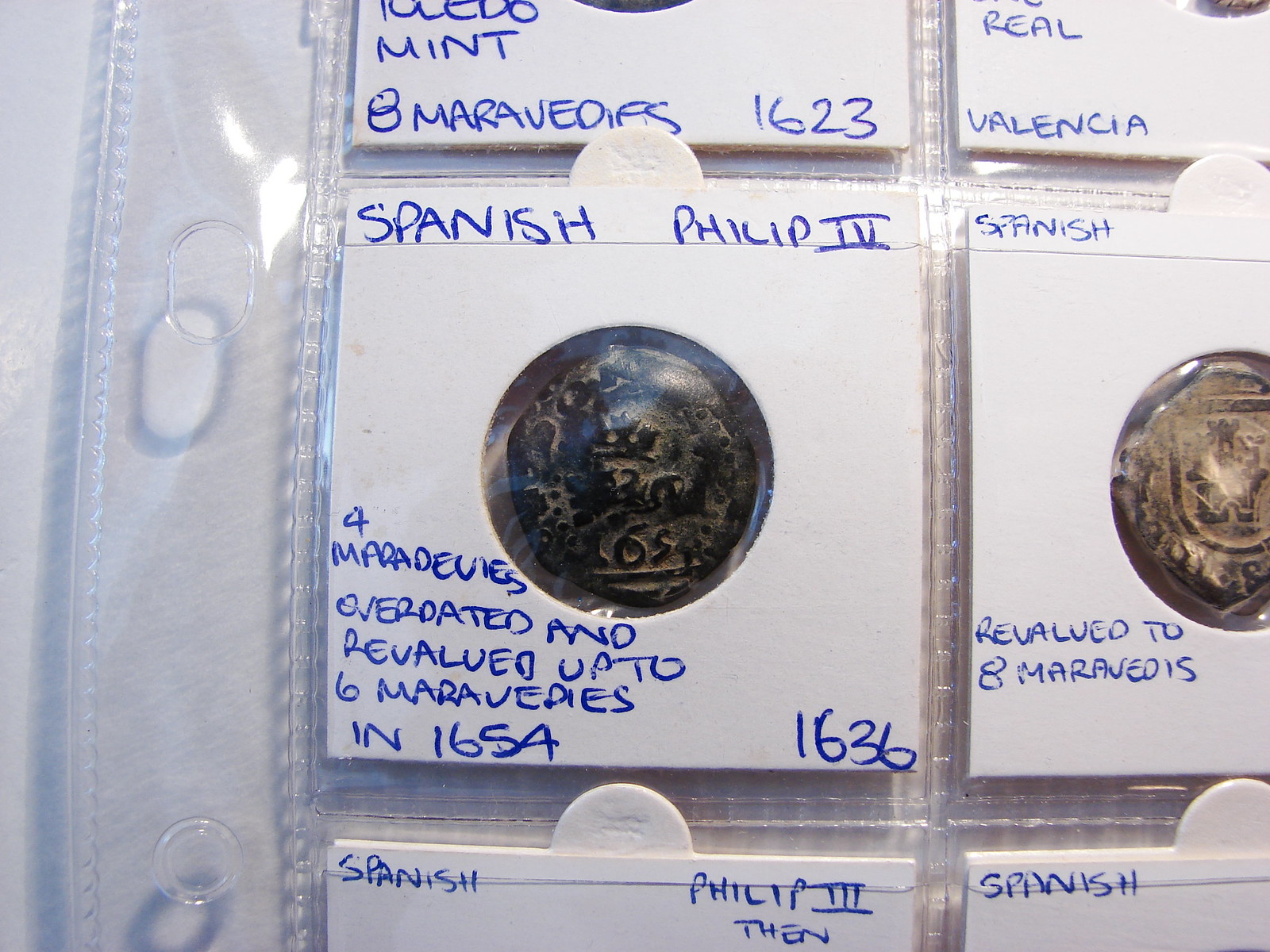The image is a colored photograph showcasing an antique coin collection, prominently featuring two coins encased in protective plastic sleeves. The plastic covers are punched for storage in a three-ring binder. One of the coins is particularly clear and labeled in blue handwritten ink, which states "Spanish Philip IV, overdated and revalued up to six maravedis, in 1654." The coin appears to be made of either bronze or copper, reflecting its significant age. Additionally, there's an indication of another date, 1636, in the bottom right corner. There are also mentions of other cropped coins – an envelope at the top and the bottom, and three more on the right-hand side. Further notes suggest the text "Spanish Philip III" below the prominent coin and another coin partially visible, indicating "Spanish."